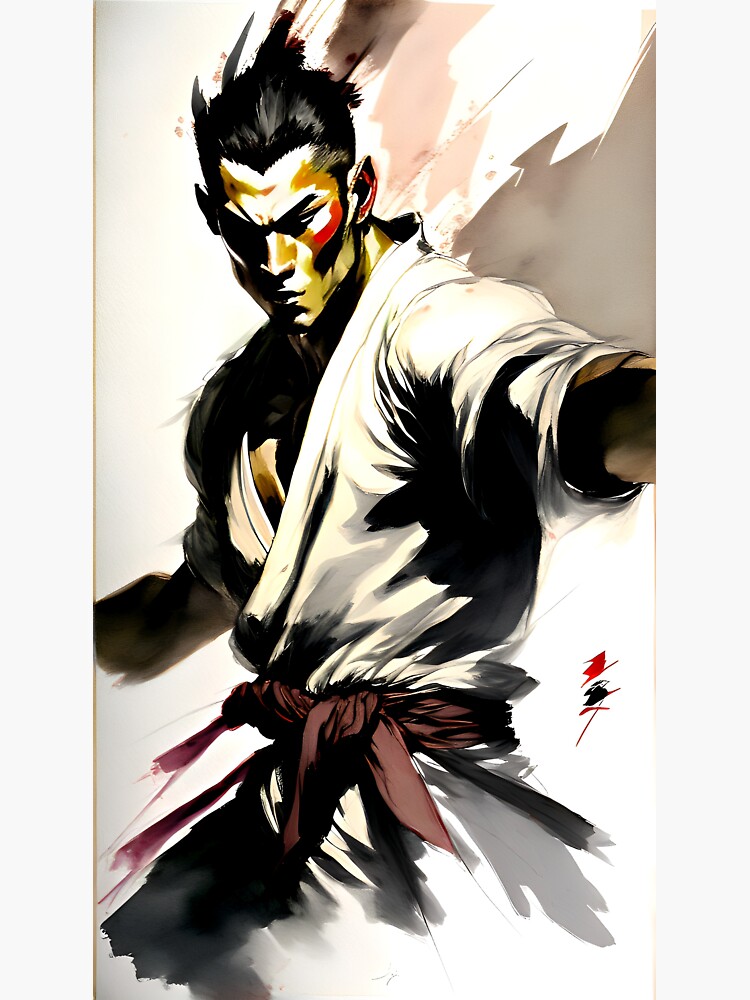This image showcases a detailed and dynamic watercolour artwork of a martial artist, possibly a warrior, characterized by his muscular build and intense demeanor. Clad in a white martial arts robe, his outfit is secured by a maroon belt tied around his waist. This warrior, with his black hair and black eyebrows, has pointy ears and a medium complexion. His facial expression is stern and angry, accentuated by a red mark on his cheek and red and black paint streaks beneath his eyes. In the artwork, his right arm is extended as if mid-punch, although his legs are not visible. The background is a mix of subtle shadows, with hues of brown, white, and orange streaks that enhance the depth and drama of the scene. Near the man's waist, red and black marks suggest signatures, adding an element of authenticity to the piece.